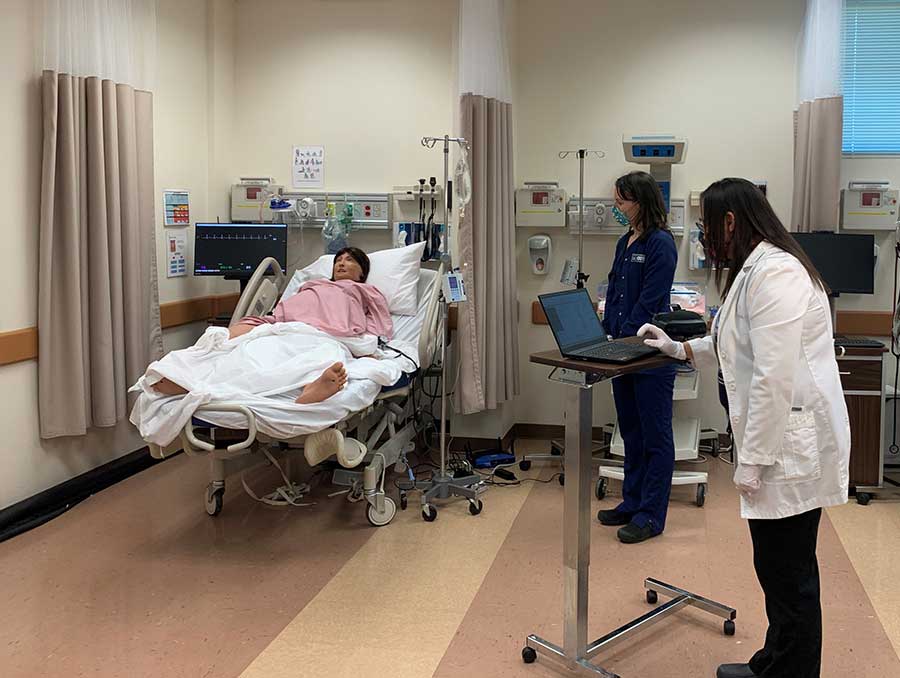In this detailed photograph, the scene is set in a hospital recovery ward with an off-white backdrop and a tiled floor of dark pink and yellow hues. The setting features divided private room sections separated by tan or brown curtains. Centrally, a lone hospital bed, adorned with white sheets and blanket, holds a patient dressed in a pink nightgown who bears a strikingly artificial appearance, suggesting this might be a training scenario. The patient, who has short black hair, is connected to various medical devices, with some kind of tool on their arm. 

To the left of the patient, on the wall, is an array of medical equipment. Meanwhile, the right side of the image shows a doctor in a white coat, wearing gloves and a facemask, working on a wooden laptop stand with a metal arm, which is adjustable in height. The doctor is intent on the screen, conveying a sense of focus. Clad in black pants and shoes, the doctor contrasts with a nurse who is positioned further back, also masked, donning a full blue outfit along with matching shoes. The overall atmosphere feels clinical and meticulously arranged, with subtle details such as unreadable text on a wall poster and the concerned expression of the patient adding depth to the scene.